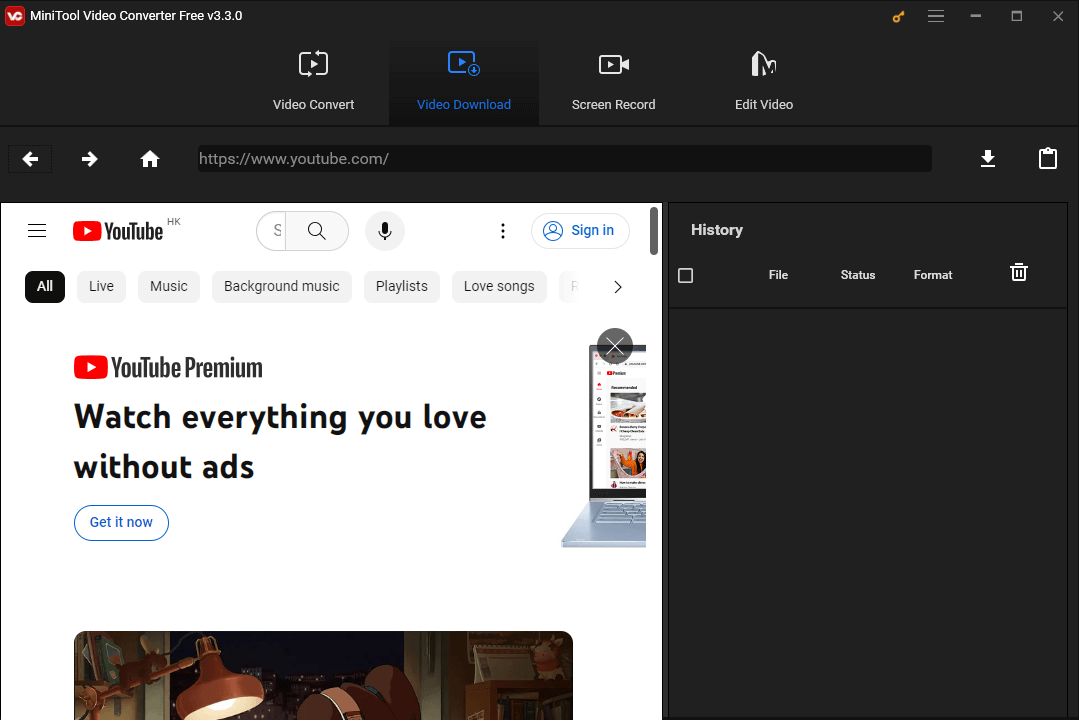The image is a screenshot of the MiniTool Video Converter Free Version 3.3.0 interface, specifically showcasing the 'Video Download' feature. This application offers four main functionalities, as indicated by the options listed at the top: 'Video Convert,' 'Video Download' (currently selected), 'Screen Record,' and 'Edit Video.' The predominantly black-themed interface features a section linked to YouTube within the app. This section displays the YouTube homepage, showing various categories such as 'All,' 'Live,' 'Music,' 'Background Music,' 'Playlists,' 'Love Songs,' and more. 

In the upper right corner of the YouTube section, the 'Sign In' button is visible, while the upper left corner shows 'YouTube HK,' indicating the YouTube Hong Kong platform. To the right side of the app, there is a 'History' pane, also in black, which is currently empty, signifying no past activities. Adjacent to the history pane, a small embedded browser window displays the YouTube website.

This detailed organization within the app allows users to easily convert, download, and screen record YouTube videos, while also providing editing capabilities. The layout is streamlined for user convenience in video viewing and downloading activities.